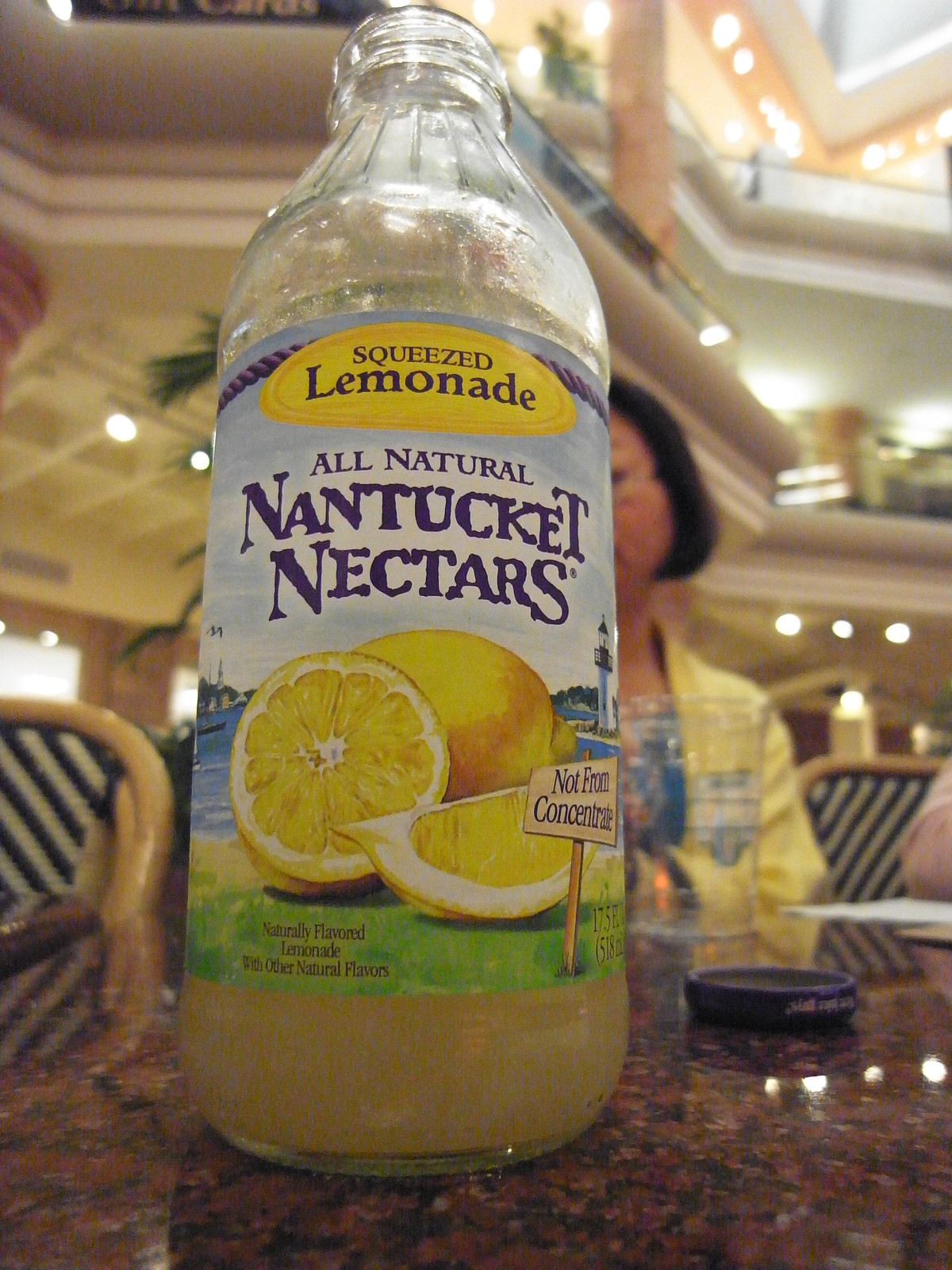This image captures a detailed scene centered around a bottle of all-natural Nantucket Nectars squeezed lemonade. The bottle, made of clear glass and partially drunk, features a multifaceted label with blue and dark blue colors, an oval yellow-orange shape, and text that reads "squeezed lemonade," "all-natural Nantucket Nectars," "not from concentrate," and "naturally flavored lemonade with other natural flavors." The label also includes an illustration depicting lemons, a lighthouse, a grassy area, and a wooden picket sign.

The bottle sits on what appears to be a marble-like plastic table situated in the food court of a shopping mall. Visible in the background are multiple levels of the mall, interspersed with plants. The scene includes an ashtray on the table, suggesting it might be an older photograph. A woman in a yellow jacket, partially visible and slightly out of focus, sits behind the bottle, adding a human element to the busy and layered background. Adjacent to the table, there are wooden chairs adorned with black-and-white striped cushions, providing a sense of casual dining ambiance in the mall.